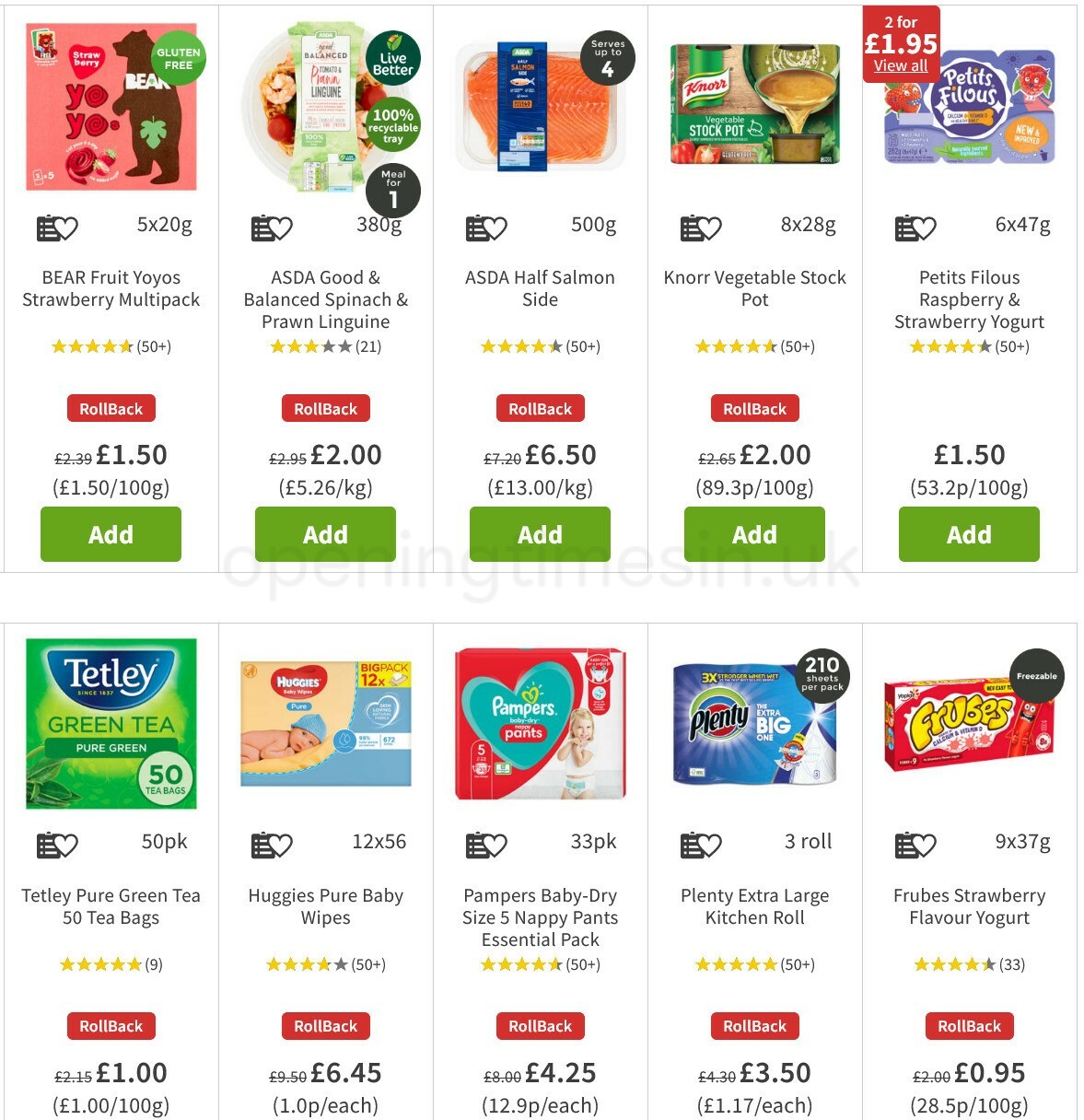This is a detailed grocery advertisement from Walmart showcasing various discounted items:

- **Fruit Yo-Yos, Strawberry Multi-pack**: Reduced to £1.50 in a rollback promotion.
- **Good and Balanced Spinach and Prawn Linguine**: Priced at £2.00.
- **Half a Salmon Side**: Available for £6.50.
- **Knorr Vegetable Stock Pot**: Priced at £2.00.
- **Petite Falafel**: Purchase includes Raspberry and Strawberry Yogurt, also at £1.50 each; buy two for just £1.95.
- **Tetley Tea**: Available for £1.00.
- **Huggies Pure Baby Wipes**: Priced at £6.45.
- **Pampers Size 5 Nappy Pants**: 33-pack available for £4.25.
- **Plenty Extra Large Kitchen Roll**: Available for £3.50.
- **Additional Yogurt Varieties**: Priced at 95p each.

This ad highlights a variety of household essentials and food items available at discounted prices.